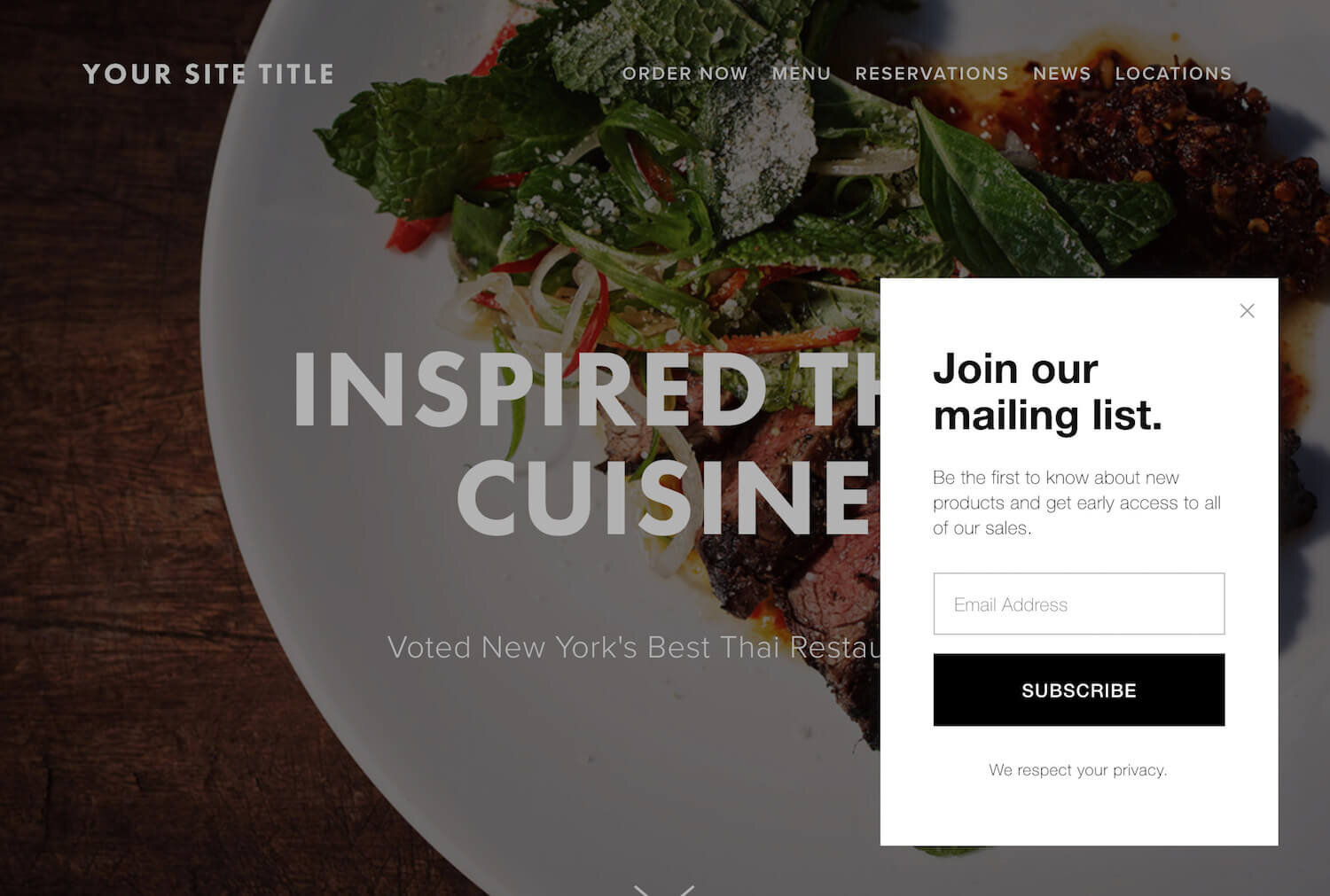A screenshot of an incomplete website dedicated to a Thai restaurant. The header prominently displays a placeholder text, "Your Site Title," indicating that the site owner has yet to finalize the design. A banner showcases a tantalizing photograph featuring a plate of beef, vegetables, and other enticing garnishes on a wooden table, with the overlay text reading "Inspired Thai Cuisine. Built in New York's best Thai restaurant." 

At the top of the page are navigational links in white font: "Order Now," "Menu," "Reservations," "News," and "Locations," allowing users to explore different sections of the site. A pop-up window interrupts the main content, inviting visitors to "Join our mailing list," with a field for entering an email address and a "Subscribe" button. The website overall appears to be in the production stage, with crucial details and customizations pending completion.